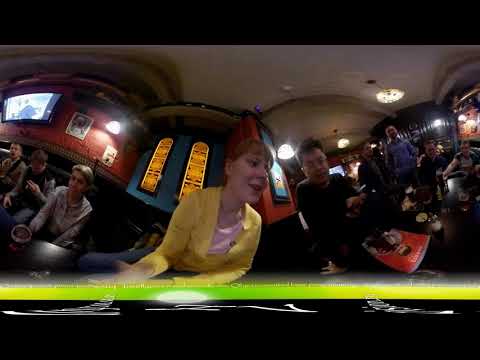The image depicts a busy indoor setting that likely combines features of a bar, restaurant, and casino, enhanced with a VR-like 360-degree perspective that creates noticeable distortions. In the forefront stands a woman wearing yellow, who appears warped due to the vantage point, with her figure stretched across both sides of the image. To her left, there are people seated at a table, engaged in conversation. On the right side, some individuals are standing, with at least one person intently focused on the woman in yellow. The bottom of the image is marked by a lime-green bar with yellow on it and distorted text, giving a digital effect. Behind them, the scene includes red brick walls, church-like stained glass windows, and ceiling lights, all contributing to the ambiance of a bar or casino. There is also a TV mounted on a wall and a possible magazine resting on a table on the right. The entire scene has an immersive quality, as if taken through a 360-degree camera.